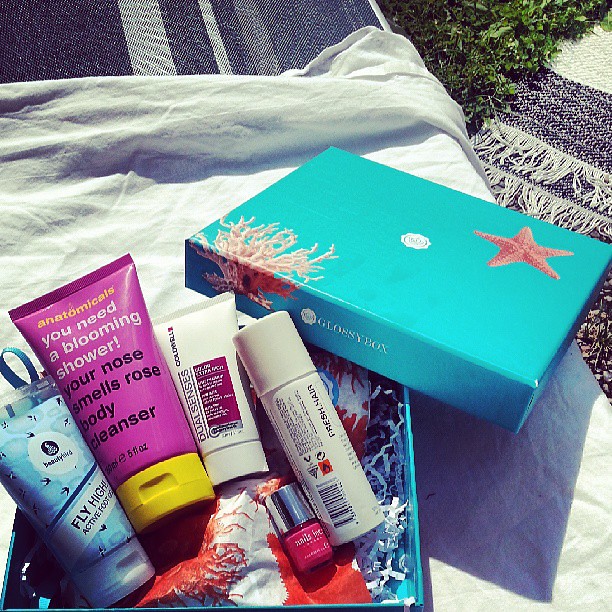This image is a detailed and vibrant product photograph capturing an open blue gift hamper box filled with various personal care and grooming items. The box, labeled "Glossy Box" on the side, is adorned with a lid featuring a starfish and coral reef design, along with the brand's circular logo. The hamper is displayed on a fringed white cloth over a grey and white patterned surface, evoking a beach-like atmosphere complemented by greenery in the background and a light-to-dark blue gradient.

Inside the box, the items are neatly arranged in a fanned-out fashion, resting on shredded paper. Prominently featured is a blue tube labeled "Beauty Bird Fly High Active Foot Cream" decorated with bird illustrations. Next is a pink tube with a yellow cap that reads, "anatomicals You Need a Blooming Shower Your Nose Smells Rose Body Cleanser." Another significant item includes a smaller white tube inscribed with "Dual Senses Colorful" within a maroon box, though finer text is unreadable. Additionally, there's a red fingernail polish bottle with a silver cap and the partial label "nail sword," and a container that appears to be either a deodorant or shampoo with "Fresh Hair" among other product details. The scene is completed with blue and white striped rugs in the foreground, enhancing the overall aesthetic of a well-curated, care-themed photo.